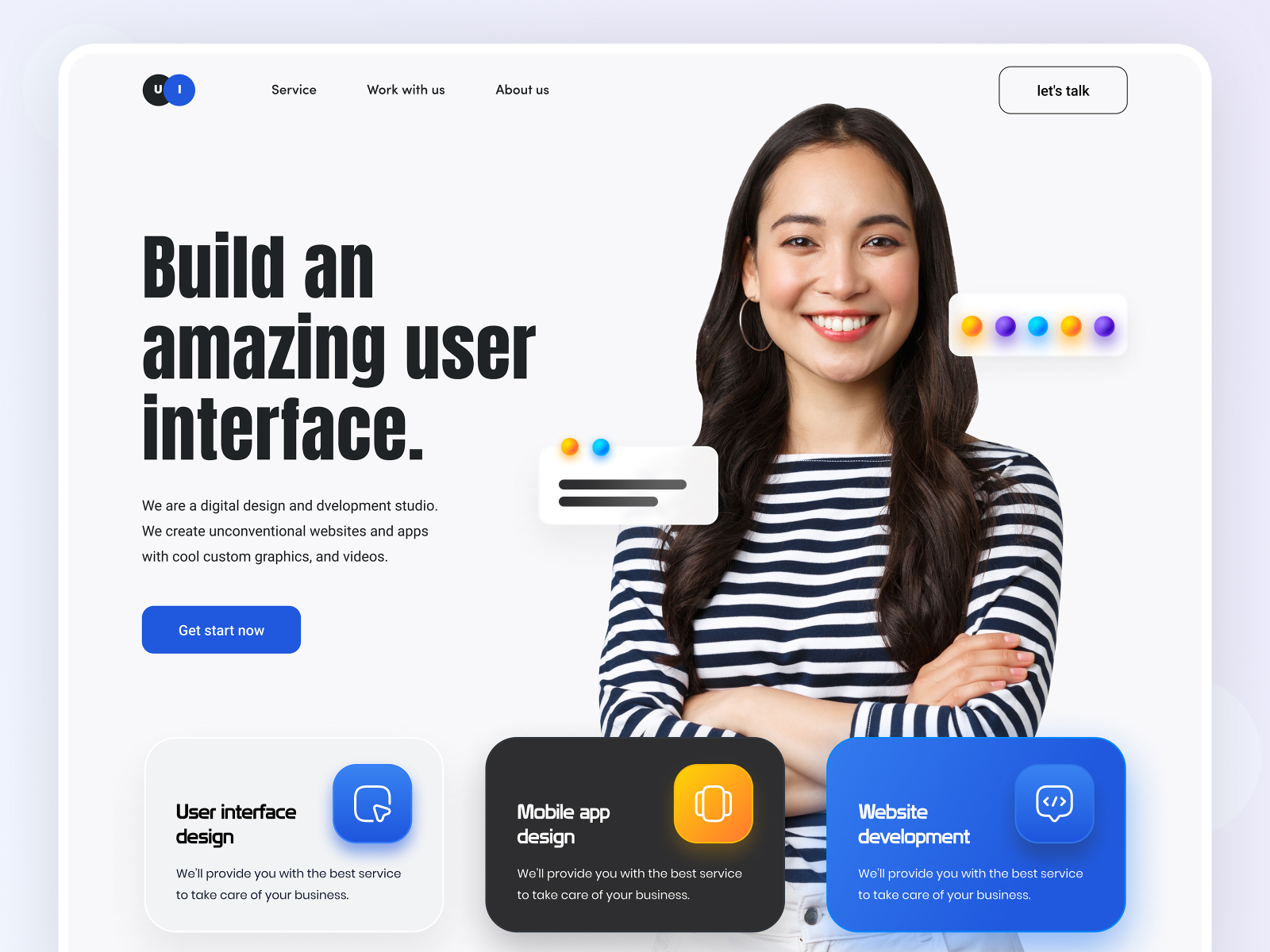In the upper left corner of the image, there are two letters, "U" and "I," displayed in white font within individual circles; the "U" is set against a black circle, while the "I" is in a blue circle. To their right, a horizontal list reads "Service," "Work With Us," and "About Us," followed by a "Let's Talk" button located on the upper right-hand side. Below this, on the right side of the image, a woman with black and brownish hair is smiling. She is dressed in a black-and-white striped long-sleeve shirt and has her arms crossed in front of her. 

The lower part of the image is divided into two sections. The left side showcases the phrase "Build an amazing user interface" with a blue "Get Started Now" button below. Directly beneath this, a smaller block titled "User Interface Design" promises the best services to take care of your business. To the right, two blocks are labeled; the first one reads "Mobile App Design," and the one adjacent to it says "Website Development."